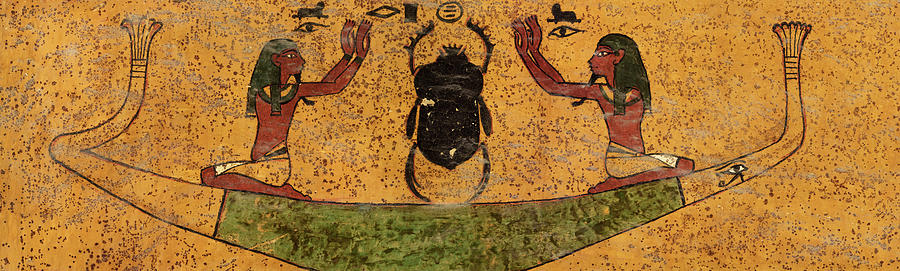The image depicts a vibrant scene from what appears to be Egyptian art, set against a gold background. Central to the scene is a large, prominent black scarab beetle, positioned between two human figures who are each kneeling at opposite ends of a U-shaped, green boat with gold ends. These figures, adorned only in loincloths and sporting beards and long hair, are depicted raising their hands in a gesture of reverence toward the beetle. Noteworthy details include the eye of Horus painted on the prow of the boat, and various hieroglyphics above the scarab, including a circle with three horizontal lines, triangles, and stylized eye symbols. The boat itself features a raised prow with leaf motifs, highlighting the rich symbolism typical of Egyptian tomb art.